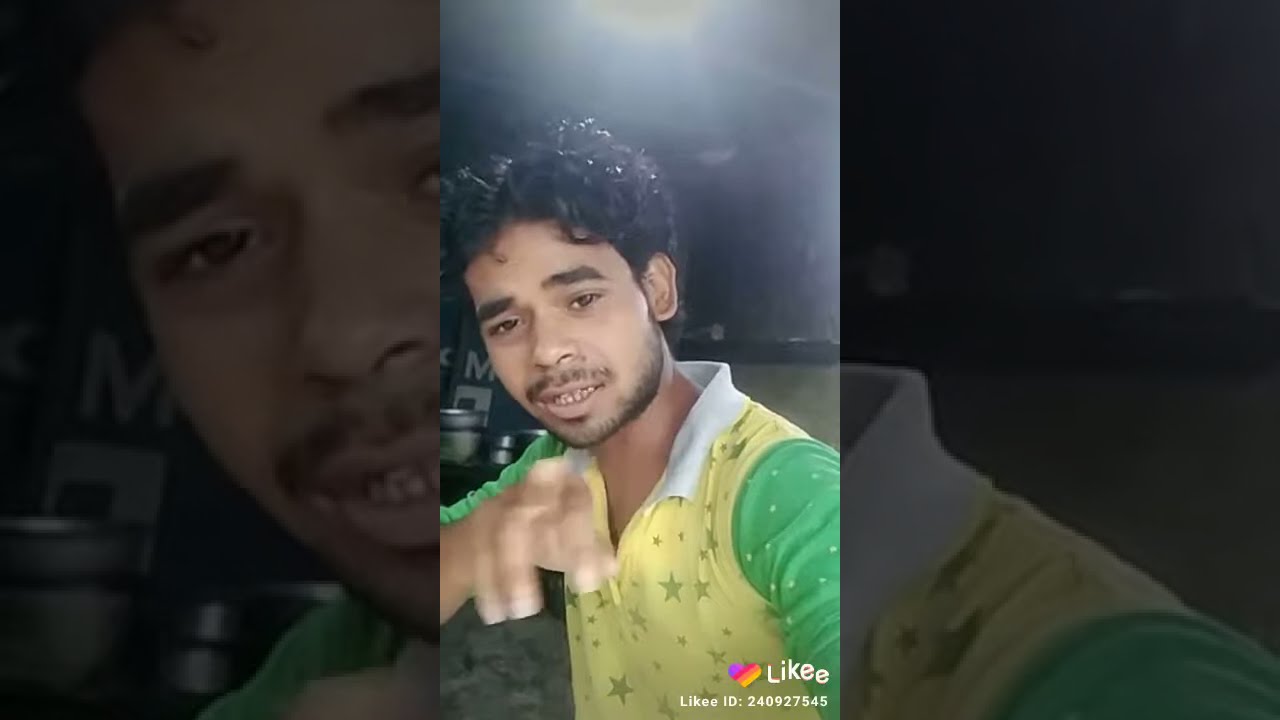In this detailed image description, we see a young man of likely Indian descent, appearing to be in his late teens or early twenties. He is captured in what seems to be a vertical video screenshot. Central to the image is a lighter, more zoomed-out view of the man, framed by darker, more zoomed-in and blurred sections on both the left and right. These sections focus closely on different parts of his face and shoulder. 

The young man has short, curly black hair, thick black eyebrows, brown eyes, and a thin mustache and beard. His facial hair is scruffy, and his mouth is slightly open as if he might be speaking. He is pointing towards the camera with his right hand, extending his index and middle fingers. 

He is wearing a distinctive yellow and green polo shirt. The main part of the shirt is yellow and adorned with gray or silver stars, while the green sleeves feature a polka dot pattern. The shirt has a white V-neck collar.

In the bottom right corner of the image, there is a colorful heart icon with stripes of purple, pink, orange, and yellow that says "LIKEE" in white letters. Below this heart icon, the text "LIKE ID: 240927545" is visible. The overall composition presents the young man in a dynamic and slightly playful posture, as if actively engaging with an audience through the camera.